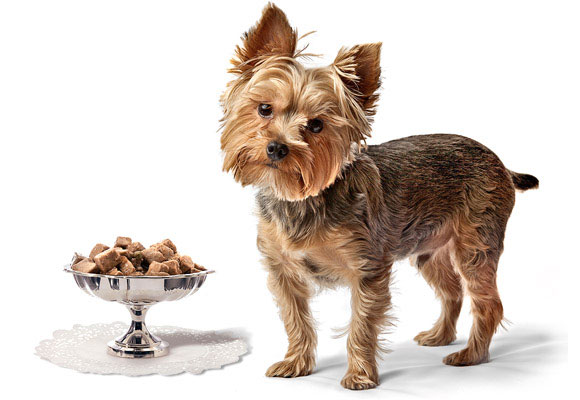This finely illustrated image showcases an adorable Yorkshire Terrier, characterized by its recently groomed body and its endearingly shaggy face. The Yorkshire Terrier, affectionately known as a Yorkie, exhibits a tan-brown and darker body fur combination, with its short, brown ears perked up inquisitively. Its black nose and beady eyes add to the charm, and its head is tilted slightly to the right, as it gazes engagingly at the viewer. The illustration, set against a white background, includes a silver platter adorned with chunks of brown dog food, resting on a white doily in the lower left-hand corner of the image. The dish appears to highlight a premium dog food brand. This detailed portrayal captures not only the breed's distinct features but also the luxurious presentation of the dog food, suggesting an advertisement for high-quality pet nutrition.